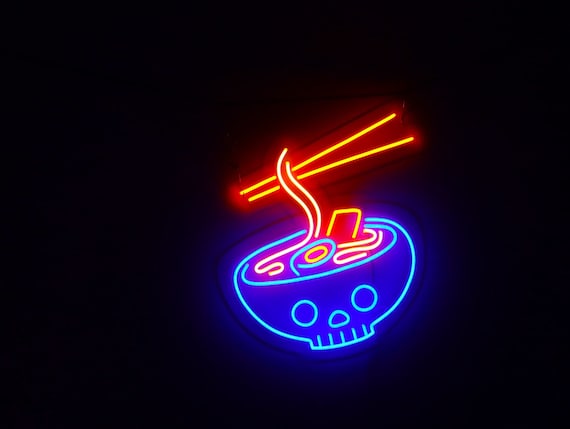The image appears to be a computer-generated or photographic representation of a neon sign set against a completely black background. The sign, located in the center of the lower right quadrant of the image, depicts a deep royal blue bowl outlined in turquoise, shaped like a skull with distinct facial features such as circle eyes, a rounded triangle nose, and horizontal lines suggesting teeth. The bowl is filled with brightly colored noodles in shades of red, blue, and yellow, giving the impression of a steaming, noodle-filled soup. Two orange diagonal bars at the top suggest steam or chopsticks lifting the noodles. The overall effect is reminiscent of a lit-up sign for an Asian noodle restaurant, offering a vibrant, artistic appeal with its neon-lit bulbs and dramatic contrasts.